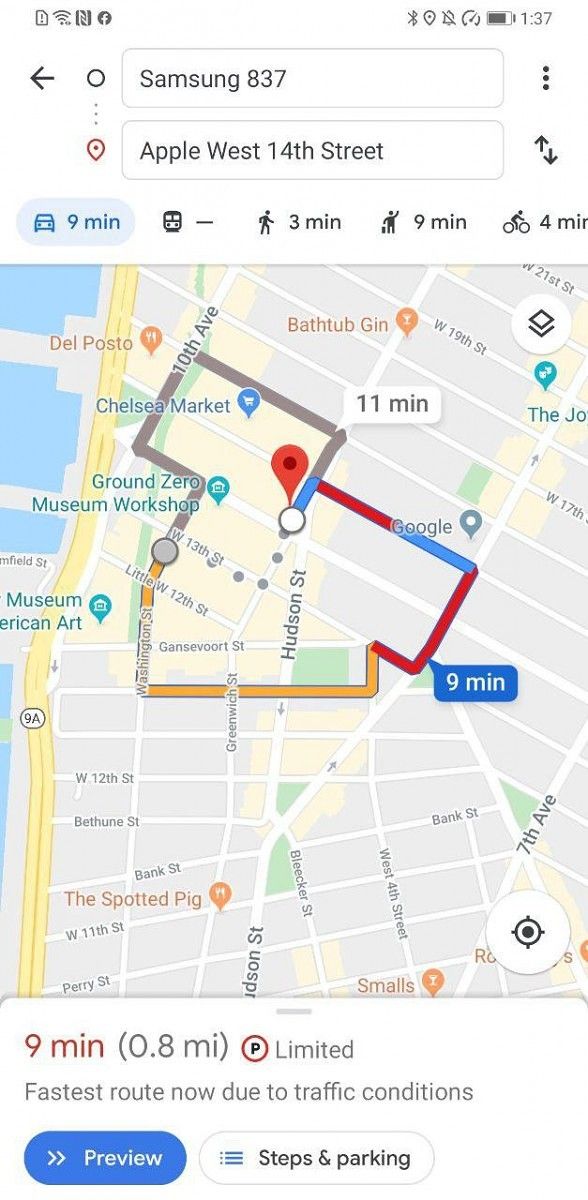Screenshot from a cell phone display at 1:37 AM or PM. The battery is at 75% capacity. Several functionalities are active, including maps, location services, Bluetooth, Facebook, and a news app, with Wi-Fi connected. The phone is navigating from "Samsung 837" to "Apple West 14th Street" using its maps application. Travel time details indicate a 0.8-mile distance, taking nine minutes by car due to traffic conditions or a brief three-minute walk. The map provides a detailed route, emphasizing the proximity between the locations.